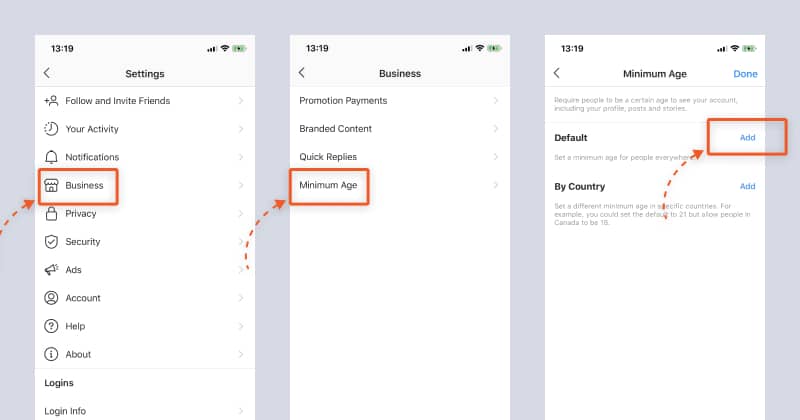The image contains three consecutive screenshots set against a gray background, each resembling a mobile phone interface. 

**First Screen**: The top-left corner displays the time "3:19" while the top-right shows a Wi-Fi signal and battery icon. The central header reads "Settings." Below this header, a list of options is presented vertically: "Follow and Invite Friends," "Your Activity," "Notifications," "Business," "Privacy," "Security," "Ads," "Account," "Help," "About," "Logins," and "Login Information." Importantly, "Business" is highlighted with an orange rectangle and an orange arrow pointing towards it, indicating a focus on this section.

**Second Screen**: The time in the top-left is now "13:19," and the same Wi-Fi and battery icons are in the top-right. The header reads "Business," presenting another vertical list of options: "Promotion Payments," "Branded Content," "Quick Replies," and "Minimum Age." The "Minimum Age" option is emphasized with an orange rectangle and an orange arrow, denoting a specific selection.

**Third Screen**: The header states "Minimum Age," with the time "13:19" in the upper-left corner, and the Wi-Fi and battery icons in the upper-right. Next to the "Minimum Age" title, there is a "Done" option. The screen shows two choices vertically: "Default" and "By Country," each accompanied by an "Add" button. The "Add" button next to "Default" is highlighted with an orange rectangle and an orange arrow, indicating it as the point of interest.

Each screen incrementally zooms into more detailed settings, with the emphasis on specific highlighted options guided by orange rectangles and arrows.